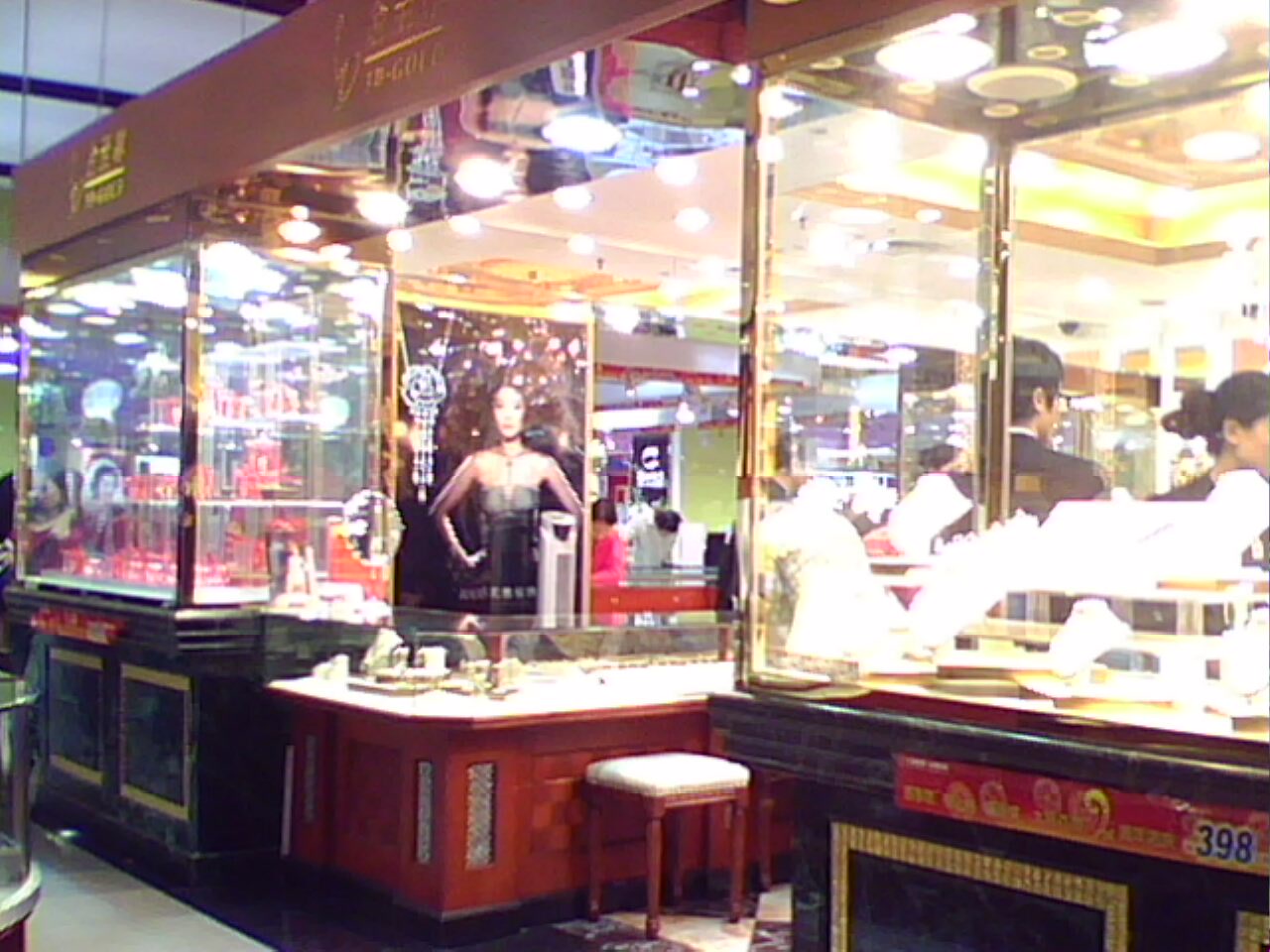This color photograph captures an indoor scene, likely taken within a mall, showcasing what appears to be a jewelry store or kiosk. The store features expansive glass windows adorned with gold trim atop black walls, allowing a glimpse into its interior despite the reflective glare. Dominating the center foreground is a poster of an Asian woman wearing a bustier-style top and a diamond necklace, with a dark background accentuating the jewelry she models. Next to her, a pair of numbers in blue, 3-9-8, stand out in the bottom-right corner of the storefront.

Inside the store, visible through the glass, are several people of Asian descent, including a man in a black blazer with a white collar and glasses, and a woman with dark hair pulled back into a bun, dressed in a dark shirt. The store's decor prominently features red and gold elements, including shiny red walls with Asian writing and a red stool-seated area with a white cushion. The overall aesthetic is bright and reflective, with considerable light bouncing off the glass and glossy surfaces. Details such as gold signage with indistinct lettering atop the storefront and boxes behind glass hint at a focus on jewelry display, reinforcing the impression that this is a high-end, possibly Asian-themed, jewelry kiosk within a bustling shopping area.